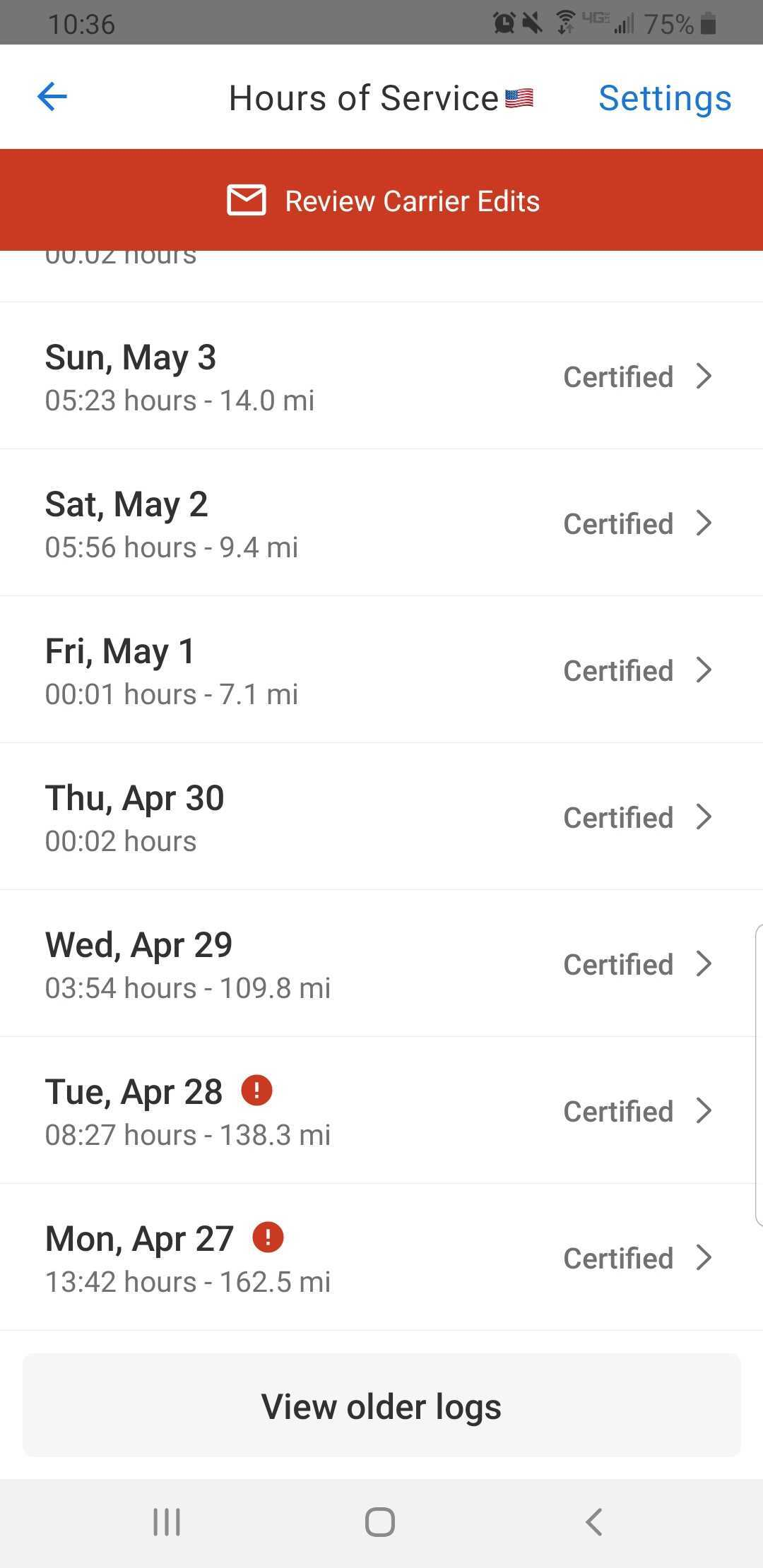Here is a detailed and cleaned-up caption for the provided image:

"A screenshot of an Android device taken at 10:36 a.m. shows the device's battery at 75%. The header reads 'Hour of Service' with a USA flag icon beside it, and to the right of that, a settings button. Below the header, there is a red message bar with a mail icon. The message, on a red background with white text, reads 'Review of Carrier Edits.' 

The main content displays a list of timestamps and certification details: 
1. Sunday, May 23, 05:20 - 05:23 hours, 14 miles certified
2. Saturday, May 2, 5:56 hours, 9.4 miles certified
3. Friday, May 1, 1 hour - 0.01 hours, 7.1 miles certified
4. Tuesday, April 30, 0.02 hours certified
5. Wednesday, April 29, 03:54 hours, 109.8 miles certified

There are two entries marked with exclamation icons:
1. Tuesday, April 28, 08:27 hours, 138.3 miles certified
2. Monday, April 27, 13:42 hours, 162.5 miles certified

At the bottom of the screen, there is a button labeled 'Reorder Log' accompanied by an Android navigation icon."